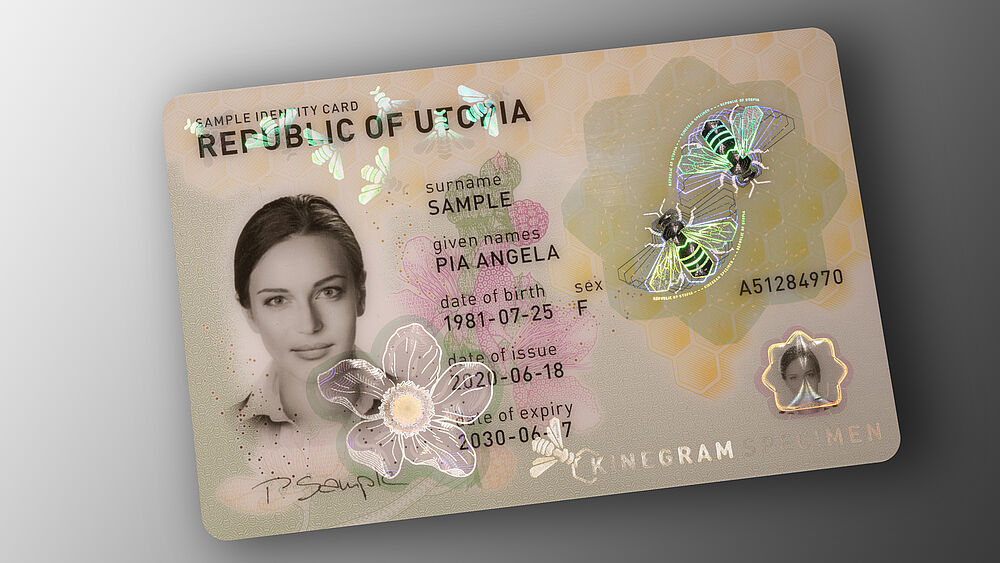This is a detailed photograph of a rectangular sample ID card from the Republic of Utopia, featuring a grey and light brown background with elegant holographic designs, including bees and flowers. The card is slightly tilted to the left, and the holographic elements create a shiny, prism-like effect across its surface. The top left corner of the card reads "Sample ID Card - Republic of Utopia." Below this, on the left side, is a black-and-white photo of a woman with her hair pulled back, wearing a collared shirt. To the right of her photograph, the card lists her surname as "Sample" and given names as "Pia, Angela," along with her date of birth (1981-07-25), sex (F), date of issue (2020-06-18), and expiration date (2030-06-17). Below her primary photo is her signature. On the right side of the card, a design pattern featuring bees encompasses a number, "A51284970," with a smaller duplicated photograph of the woman beneath it. Additionally, at the very bottom right corner, there is a logo indicating "kinogram specimen."